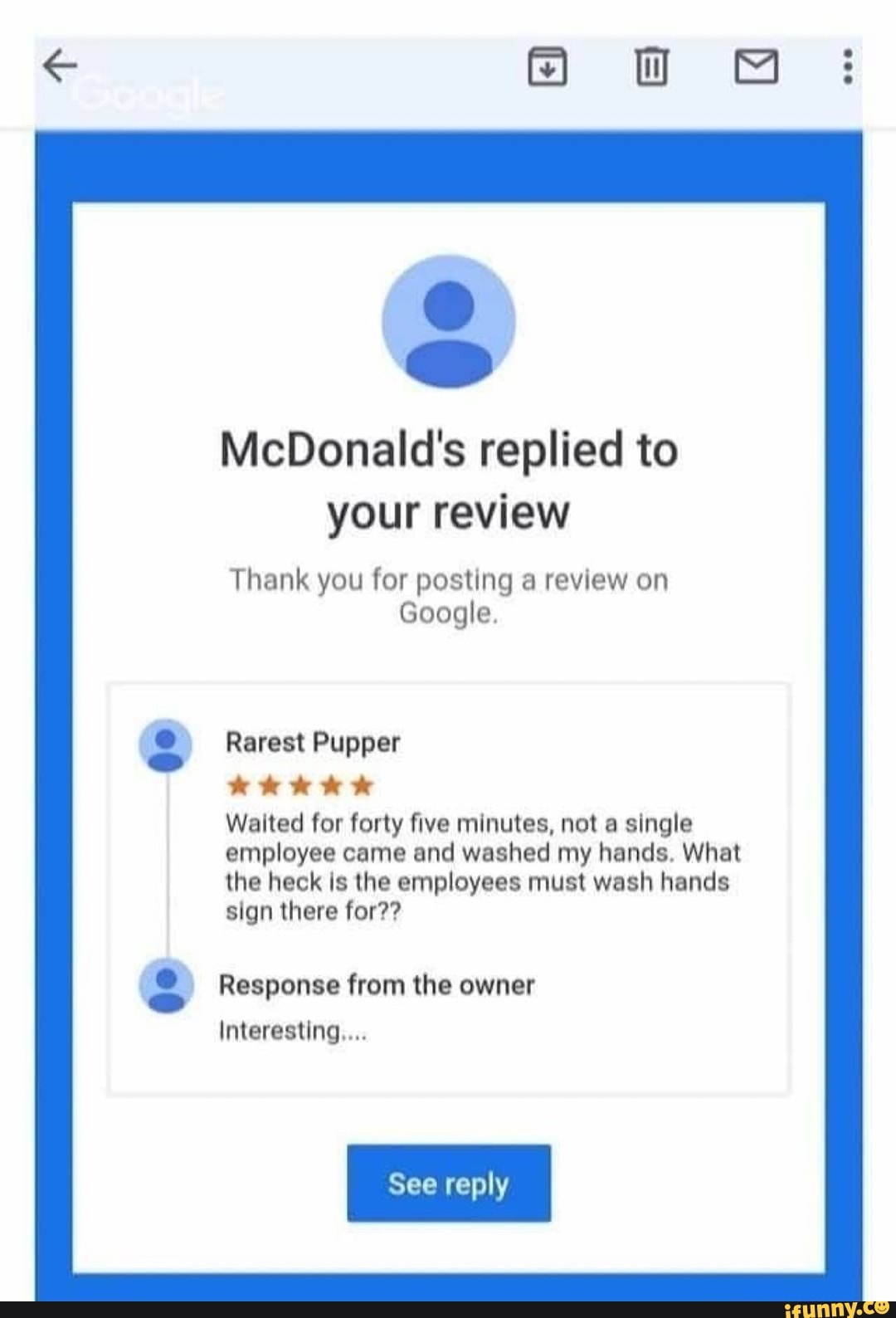**Detailed Caption:**

The image is a screenshot taken from a mail application that captures a humorous exchange between a user and McDonald's. This screenshot has a narrow, thin black banner at the bottom displaying the iFunny.co logo in bright yellow on the right side. At the top of the screenshot, a light blue banner hosts various utility icons: a grey arrow pointing left situated at the far left, followed by symbols including a trash can, a mail icon, and a three-dot menu on the right side.

The main content area of the screenshot features a white box with a dark blue border. Centered within the white box, the text reads "McDonald's replied to your review" in black lettering. Above this text is a placeholder circle resembling a LinkedIn profile photo, indicating a user’s avatar. Below the initial message, in grey text, it states, "Thank you for posting a review on Google."

Following this, the original review is displayed, attributed to a user named "Rarest Pupper" who has given a five-star rating. The review humorously complains: "Waited for 45 minutes, not a single employee came and washed my hands. What the heck is the 'employees must wash hands' sign there for?!!"

The screenshot then shows the response from the owner: "Interesting..." with ellipses marking the end. Lastly, there's a button at the bottom labeled "See Reply," prompting the user to view the full conversation on the web page.

The color contrast and layout are designed to mimic an actual mail notification, adding a layer of satire to the meme.